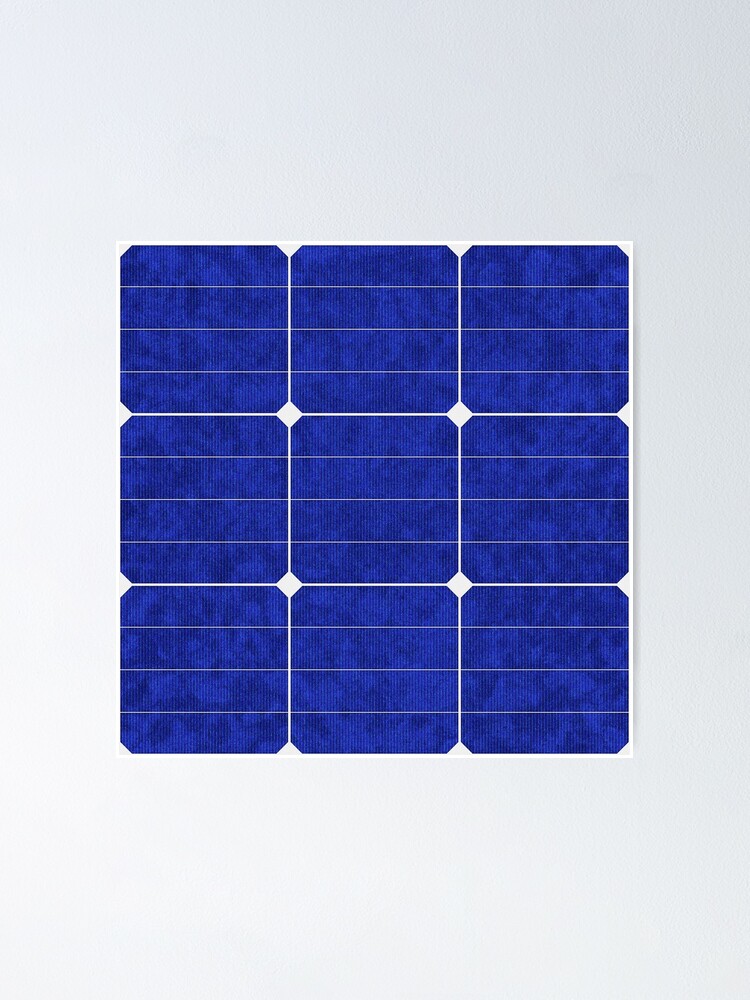The image depicts a computer-generated design consisting of nine individual squares arranged in a 3x3 grid pattern on a plain white or light gray background. Each square is a rounded or chamfered dark blue tile with hints of darker blues within, creating a varied texture. The tiles are separated by thin white lines, which sometimes give the appearance of white diamonds at their intersections. Additionally, each square features three equally spaced horizontal white lines running across it, akin to thin guitar strings or part of a grid system. These lines contribute to a sense of structure and organization within each blue tile. The overall impression is one of a meticulously crafted, abstract design, reminiscent of a modern painting or a digital art piece.